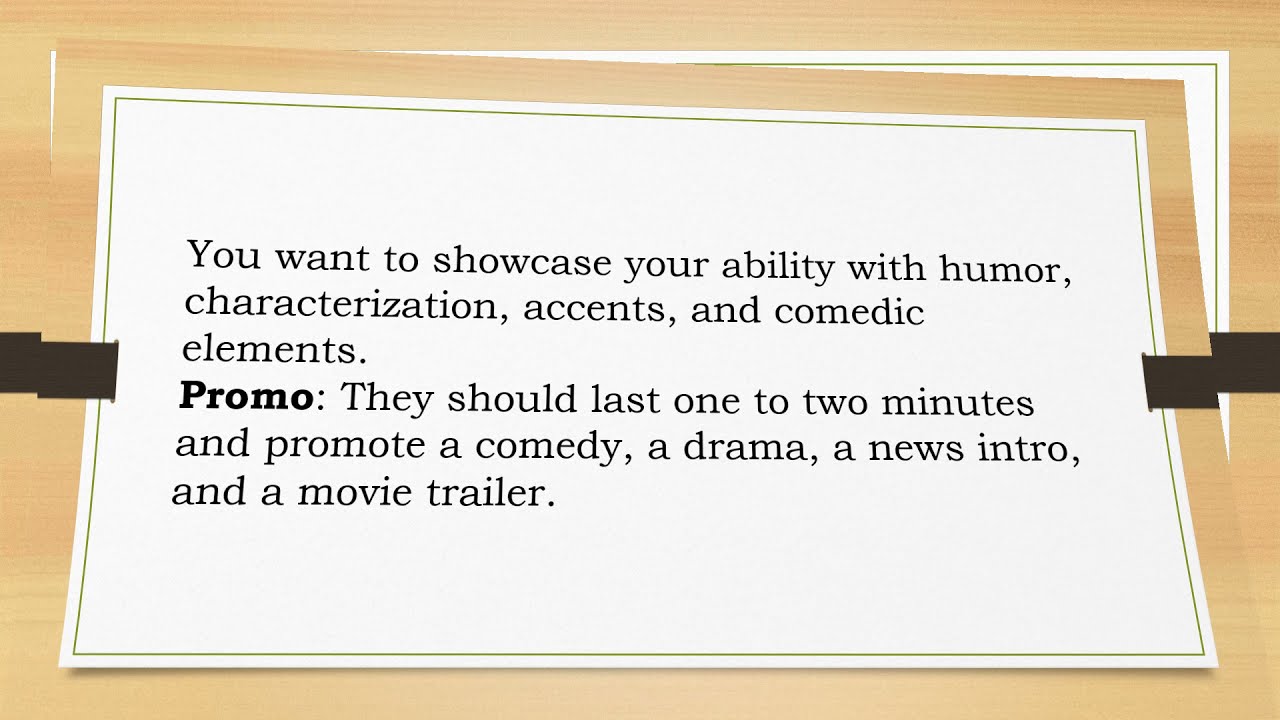This wide rectangular image displays a piece of paper slightly bent at the corners, positioned on a light brown oak-colored wooden surface. The paper, which spans most of the image, features a narrow black border framing it. On either side of the paper, there are two identical black rectangular objects inserted through small holes. The paper's text, printed in standard black font, reads: "You want to showcase your ability with humor, characterization, accents, and comedic elements." Below this, the word "PROMO" is bolded. The subsequent line, rendered in normal font, specifies, "They should last 1-2 minutes and promote a comedy, a drama, a news intro, and a movie trailer." The simple, clean design of the paper suggests it may be part of a card game or a promotional material, with its precise layout and clear instructions accentuated by the contrasting black text and white background.